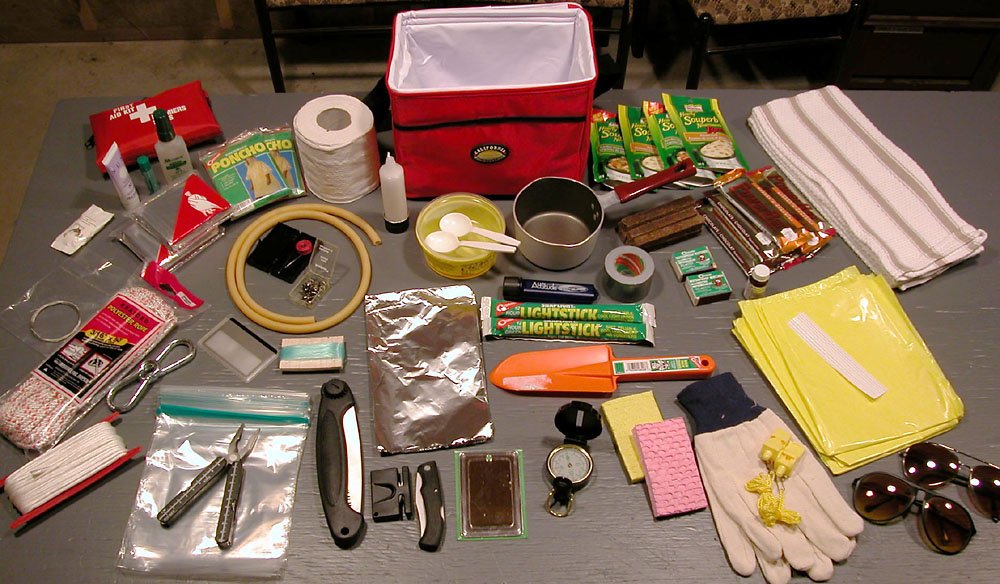The image depicts a comprehensive emergency kit laid out on a gray table. In the background, there are chair legs and a gray surface holding a red cooler. The table is filled with an extensive array of survival items commonly used for camping or emergencies. Prominently visible are a first aid kit, rain ponchos, and a roll of toilet paper. Several items seem essential for various scenarios, including multiple bottles, a length of rope, twine, a pair of snippers, a utility knife, and aluminum foil. Light sticks and an orange shovel are centrally positioned, with a green shovel-like tool nearby. A variety of other tools, including a pressure gauge, a silver metallic bag possibly containing folded knives, are spread across the table. Cleaning and utility supplies such as sponges, work gloves, and perhaps garbage bags are also present. The kit includes packets of food, a cooking pot, two spoons, duct tape, and sunglasses. Other notable items on the table are a compass, wire, fire starters, cloths, and bowls. The collection is quite diverse, containing many items whose specifics are unclear but suggest thorough preparation for various emergency or survival situations.